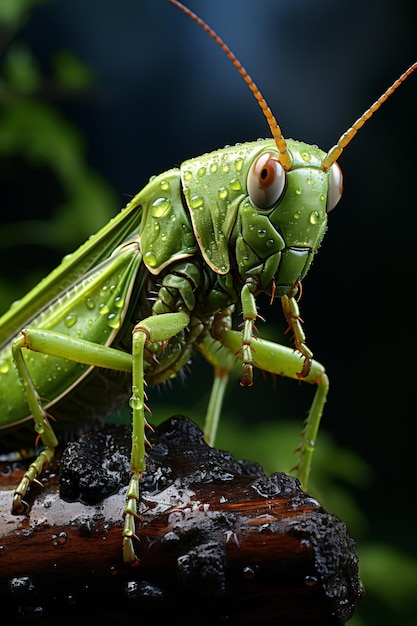This image showcases an incredibly detailed, up-close shot of a bright chartreuse green insect, resembling a praying mantis or grasshopper. The insect's body is meticulously covered in glistening dew drops, which appear almost too perfect, suggesting either an extraordinary high-quality photograph or a masterful 3D computer illustration. The mantis, with its striking red eyes and yellow-brown antennae, stands prominently on what seems to be water-rotted driftwood, although some might interpret it as a shiny black obsidian rock. The insect's positioning and the diagonal point of view make it appear as if it's staring directly at the viewer, creating an almost lifelike and immersive experience. The background is highly blurred, containing hints of green and dark blue, emphasizing the sharp focus on the insect and enhancing the overall surreal, almost hyper-realistic quality of the image.